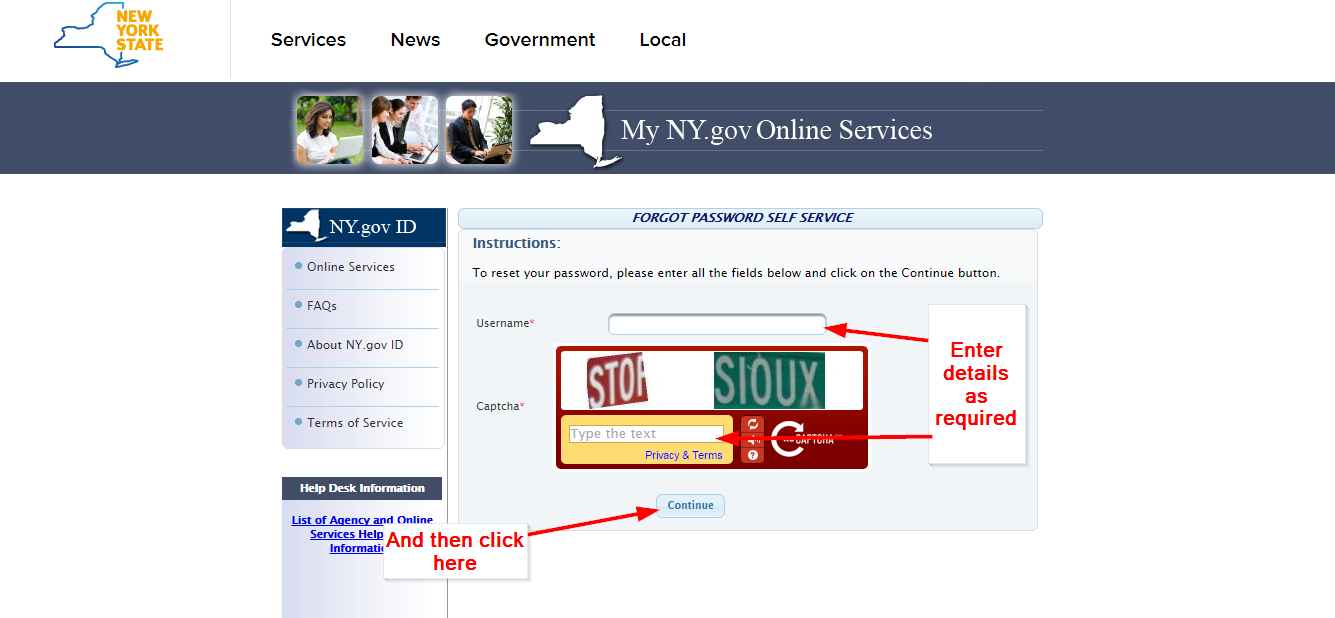This is a detailed view of a screenshot taken from the official New York State website. In the upper left-hand corner, an outline of the state of New York is prominently displayed, serving as a recognizable emblem. To its immediate right, a horizontal menu bar presents key navigation options: Services, News, Government, and Local. Below this navigation bar, the title "MyNewYork.gov Online Services" is prominently featured, indicating the section of the website currently in focus.

In the main content area on the left-hand side, a vertical menu offers additional options such as Online Services, FAQs, AboutNewYork.gov, ID, Privacy Policy, and Terms of Service. The central portion of the screen is taken up by the "Forgot Password Self-Service" page. This page provides an organized, step-by-step guide to assist users in resetting their passwords, ensuring that they can regain access to their accounts securely and efficiently. The structured layout and clear instructions exemplify the user-focused design of the website, aiming to facilitate ease of use for all visitors.